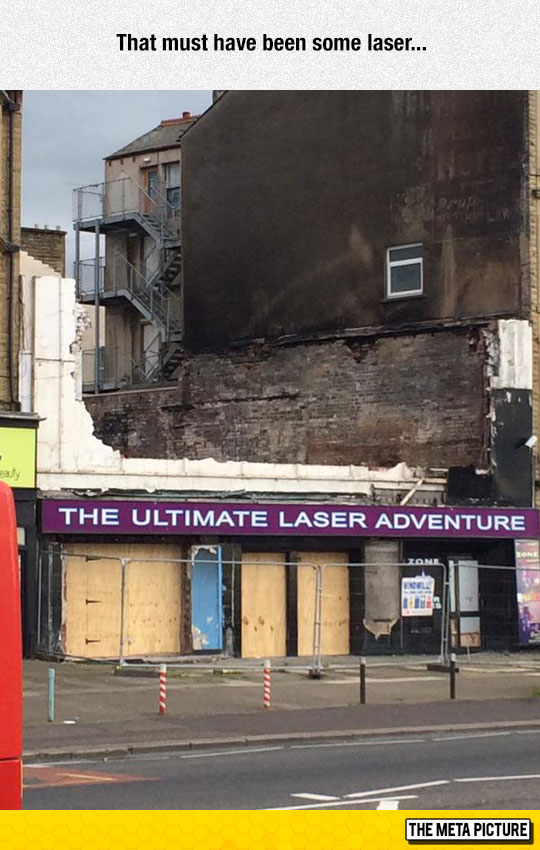This portrait-style photograph showcases a downtown scene featuring a notably distressed and abandoned building. At the bottom, the image begins with a road bordered by a sidewalk equipped with small vertical poles to prevent vehicles from crossing. In front of the building stands a fence, likely chain-link, which is difficult to see due to its transparency. The primary structure, visibly rundown, sports light brown exterior walls and has its windows and doors boarded up with plywood. A dark purple sign with white letters reading "The Ultimate Laser Adventure" is affixed above the entrance. The second floor appears completely destroyed, with remnants of scorched walls hinting at a past fire. Adjoining this building to the right is a brick building, relatively unscathed by the fire, featuring cracked and damaged areas at its base and a fire escape made of gray metal extending up three floors. The brick facade includes exposed brickwork and windows. A yellow border runs along the bottom of the image, with a white box on the right corner containing the text "the meta picture" in black font. There are no vehicles on the street, emphasizing the desolation of the scene.